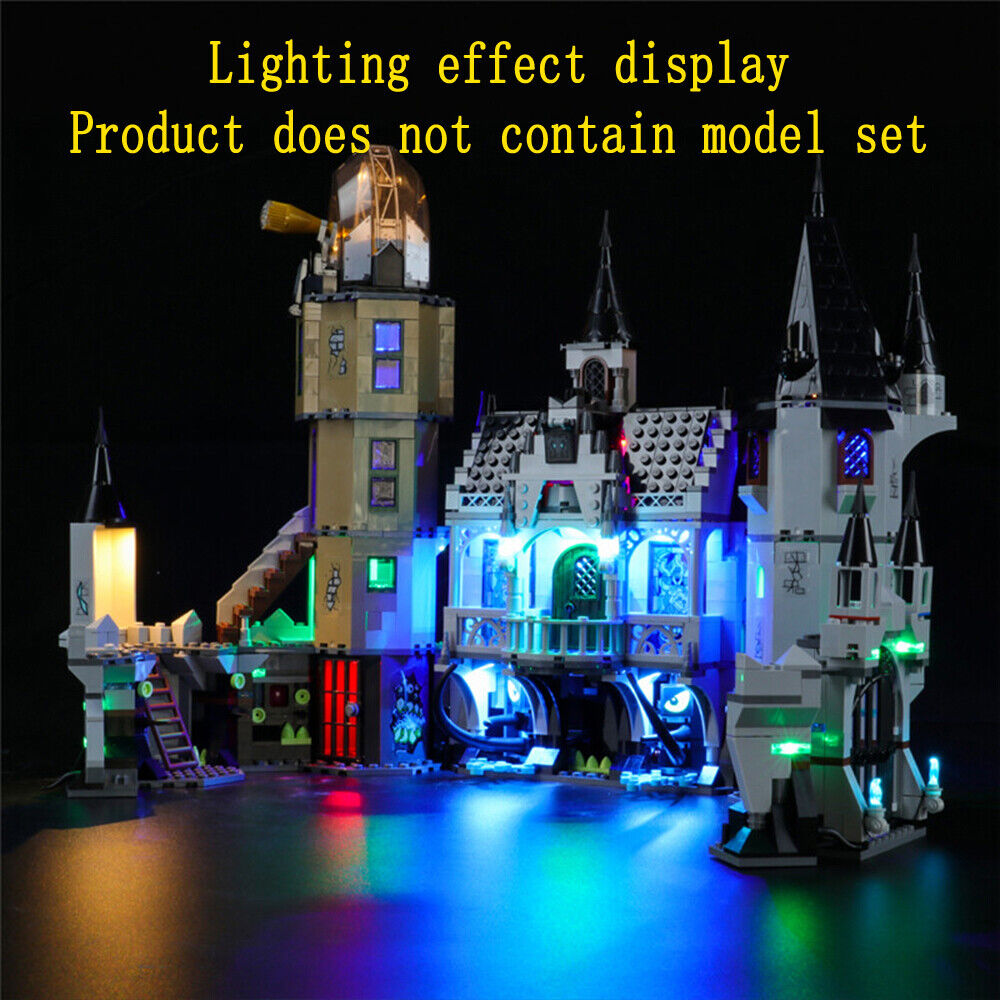The horizontal rectangular image displays the cover of a product box for lighting effects, as indicated by the yellow text at the top: "Lighting Effect Display Product Does Not Contain Model Set." Dominating the scene is a detailed model that appears to be crafted from Lego-like blocks. The model features an outdoor scene centered around a house resembling a little cottage, possibly set on the water with two boats below it. The house, characterized by a porch, a turret on the side, and a large rope extending out, is intricately designed with various lighting effects.

The top part of the model house is colored in shades of gray and blue, with a green door and prominent steps leading up to it. The entire house is illuminated primarily in blue light, which contrasts with the surroundings. There’s a balcony that adds to its detailed architecture. Adjacent to the house, a castle-like structure with pointy turrets, a lookout tower, and ladders is visible, adorned with multicolored lights. The right side of the image shows the castle with green and blue lighting, while the left turret glows yellow and the door of the tower is highlighted in red. White candelabras flank the main door, further enhancing the scene's illuminated beauty. The entire setup is placed on a shiny surface, reflecting the myriad colors of the lights, set against a completely black background that accentuates the vibrant hues of the lights.